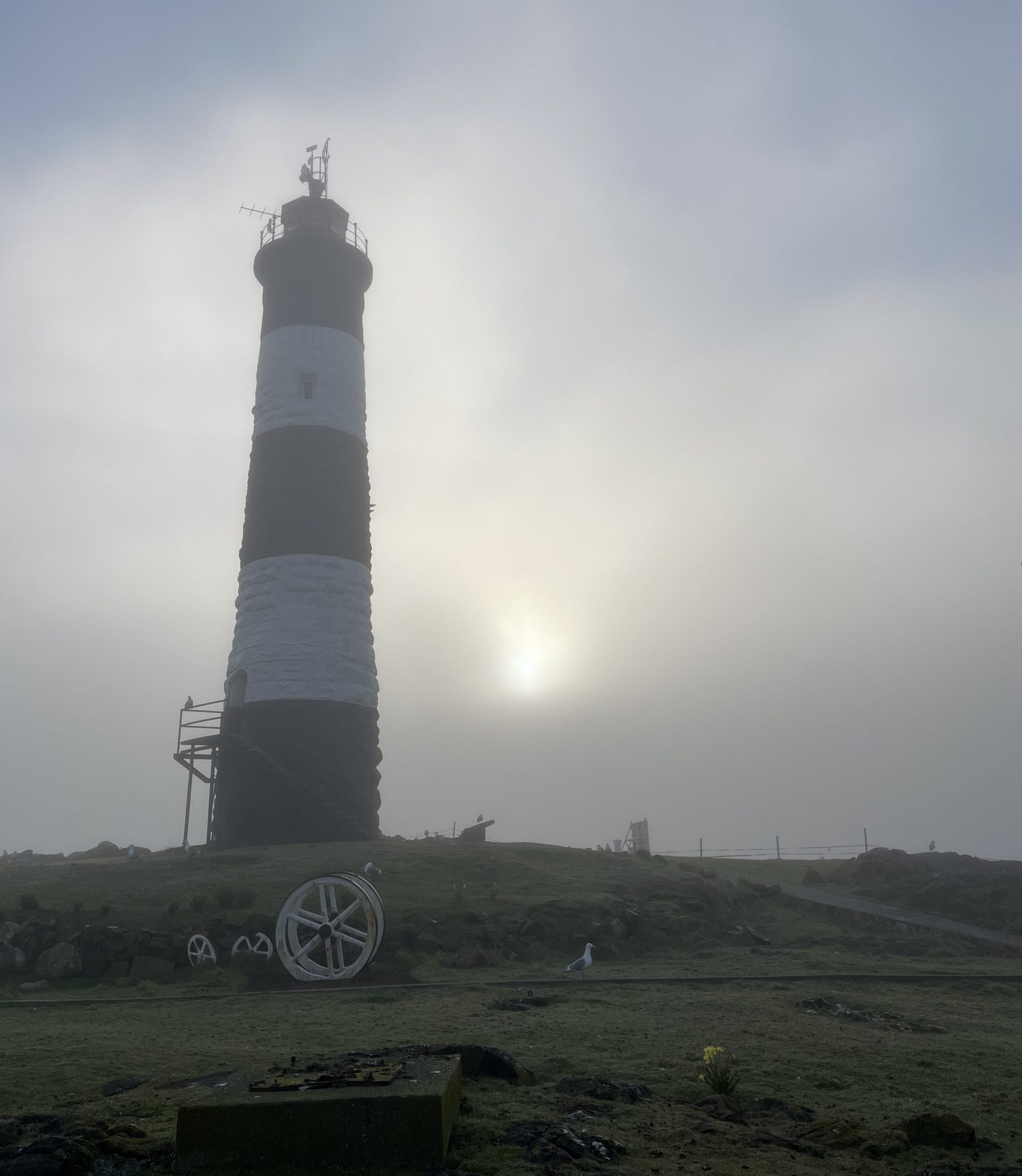This color photograph captures a foggy scene featuring a prominent lighthouse perched atop a grassy hill. The sky is hazy with a grayish fog, obscuring the ocean, but a faint glimmer of sunlight manages to pierce through the clouds. The lighthouse is striking with its alternating horizontal stripes of red and white, crowned with a metal staircase and various antennae. In the foreground, a seagull stands on a cement block amidst the tall grass. At the base of the hill, three white wagon wheels are visible, adding a rustic touch to the setting. A path winds up the hill to the lighthouse, which is fortified with a fence at the top. The image is devoid of people, allowing the viewer to fully absorb the serene yet slightly ominous atmosphere created by the fog and the solitary lighthouse.